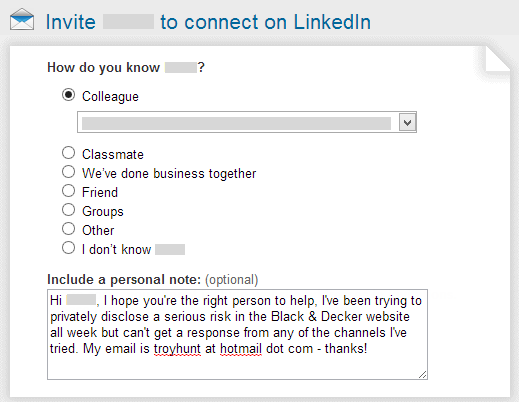A detailed caption for the image would be:

---

The image displays a screenshot of a LinkedIn invitation to connect interface. The interface features a topless envelope icon, signifying a new message or invitation. The invitation prompts the receiver to verify their connection with the sender by providing several unchecked options: "Colleague," "Classmate," "We’ve done business together," "Friend," "Groups," "Other," and "I don’t know [Name]." 

Beneath these options is a field for including a personal note, which is optional. In this specific case, the note reads: 

"Hi, 

I hope you’re the right person to help. I’ve been trying to privately disclose a serious risk in the Black and Decker website for a whole week but can’t get a response from any of the channels I’ve tried. My email is joyhunt2@hotmail.com. Thanks."

The borders of the message box are gray, and the text body is also gray contrasted against a white background. The overall layout of the LinkedIn interface captures the structured and professional format used for connecting and communicating within the platform.

---

This description clearly outlines the elements within the image and provides context to the message being sent.